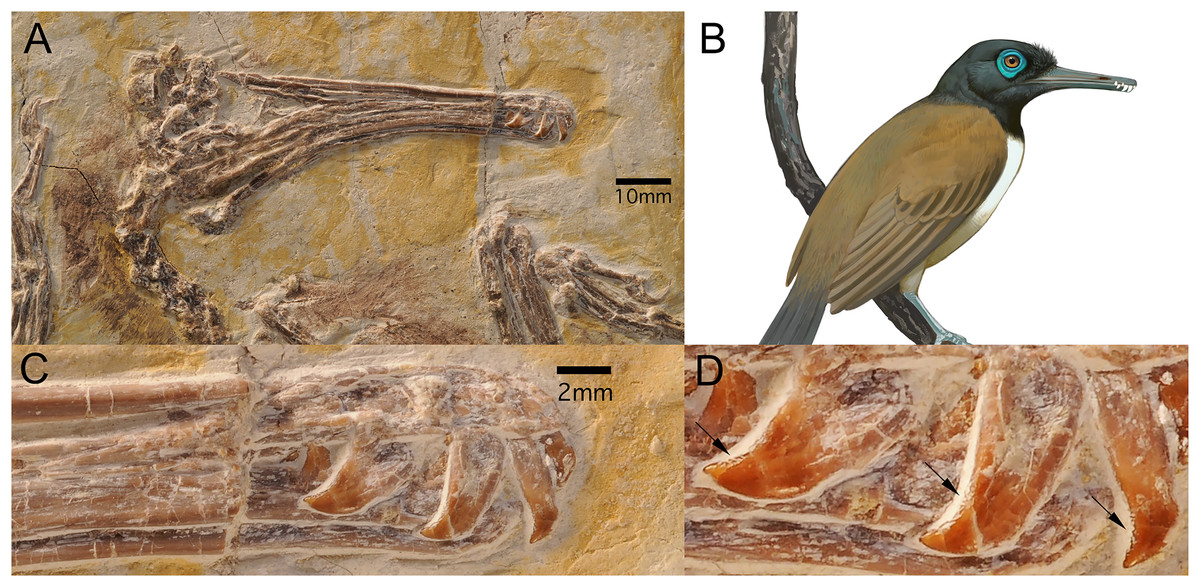The image consists of a detailed chart divided into four sections labeled A, B, C, and D, depicting a combination of fossils and digital renders. Section A, in the top left corner, shows a fossil impression on a stone wall of what appears to be a stalk of grain or flowers, marked with a size indicator of 10 millimeters. Directly below it, Section C, displays another fossil impression or carving that resembles a bear, measured at 2 millimeters. To the right, Section B presents a computer-generated image of a bird perched on a branch. This bird features a black head, a distinct blue ring around its eye, a black beak, brown wings, and a white belly, holding an indistinguishable object in its beak, possibly a bug. Finally, Section D offers a close-up view of the bear fossil's feet, highlighting specific areas with arrows pointing to the feet and showing where the image has been worn down from rubbing. The representations in the image provide a mix of natural history artifacts and digital illustrations, meticulously characterized by scale and visual detail.